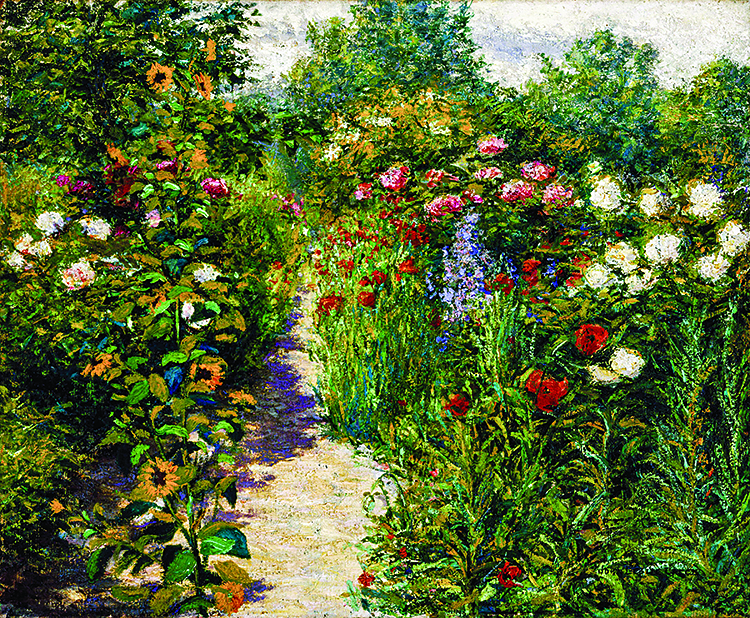A vibrant impressionist painting vividly captures a diverse field of wildflowers in a medley of lush greens, sunny yellows, delicate pinks, fiery reds, soothing blues, and pristine whites. Dominating the foreground, a sandy tan path meanders off-center towards the left, its surface dappled with the shadows cast by nearby flora. This path subtly guides the viewer's eye through the colorful disarray of nature. Among the blooms, recognizable flowers such as black-eyed Susans, clusters of white blossoms, and striking red poppies stand out, interspersed with an assortment of tall weeds and verdant leaves. In the background, a dense line of trees meets the sky, completing the serene landscape with a touch of horizon beyond the floral profusion.